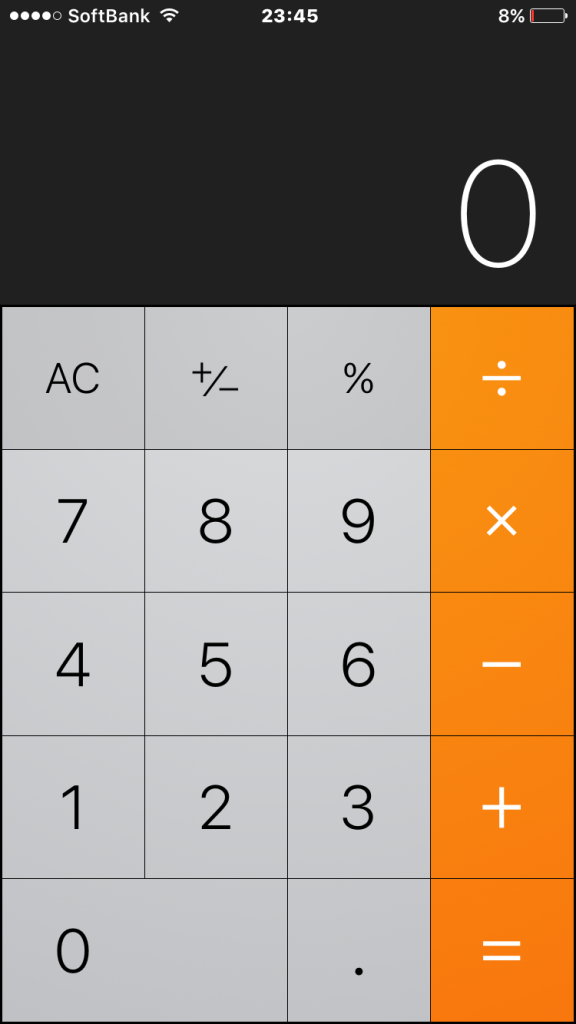The image shows a dark grey background with a calculator interface prominently displayed. In the top left corner, there is the SoftBank logo, accompanied by a signal strength indicator with five dots – four solid white dots and one hollow dot. To the right of the SoftBank logo, there is a full Wi-Fi bars icon, followed by the time "23:45". Next to the time is a battery icon indicating 80% battery life, depicted in red to show it is almost depleted.

The calculator interface below consists of 19 buttons arranged in a grid. From the top left, the buttons are as follows: 'AC', plus/minus symbol, percentage symbol, and division symbol (orange). The second row includes the numbers '7', '8', and '9', followed by the multiplication symbol (orange). The third row contains the numbers '4', '5', and '6', followed by the subtraction symbol (orange). The fourth row includes the numbers '1', '2', and '3', followed by the addition symbol (orange). Finally, the bottom row consists of the number '0', a decimal point, and the equals symbol.

All numerical buttons and the decimal point are grey, while the operation symbols (division, multiplication, subtraction, and addition) are orange, standing out starkly from the rest of the keys.